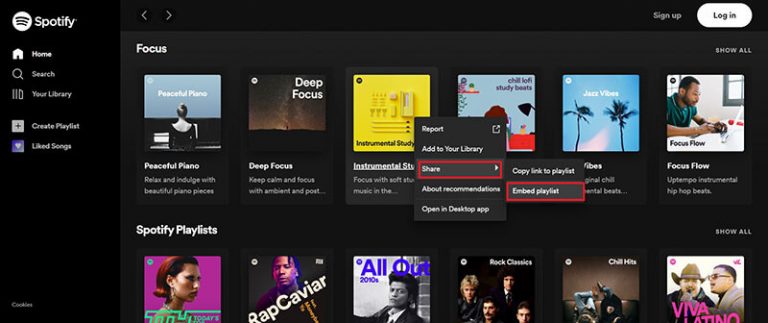The image depicts the Spotify website, a prominent music streaming service. In the top left corner, the Spotify logo and its accompanying icon are prominently displayed. Adjacent to the top right, there are options for users to either sign up for a new account or log in to an existing one.

On the left sidebar, directly below the Spotify icon, there are several navigational buttons: a home button for the main page, a search button for exploring content, and a library button for accessing the user's saved music and playlists. Following these, there is a "+" icon for creating a new playlist, and beneath that, a heart symbol labeled "Liked Songs," which likely contains tracks the user has given a thumbs up.

The right side of the interface features two distinct rows. The first row, titled "Focus," offers six playlist options designed for concentration, including "Peaceful Piano," "Deep Focus," "Instrumental Study," and "Chill." The fifth option is partially legible but seems related to "Chill," and the sixth option is "Focus Flow," which includes an image with a couple of trees in the background. One of these playlist icons appears to be selected, revealing share and embed playlist options in a dropdown.

At the bottom, a section labeled "Spotify Playlists" presents another selection of playlists. Although some of the titles are cut off and not fully readable, identifiable options include "Rock Classics," another "Chill" playlist, and a playlist likely featuring Tejano or Latino music.